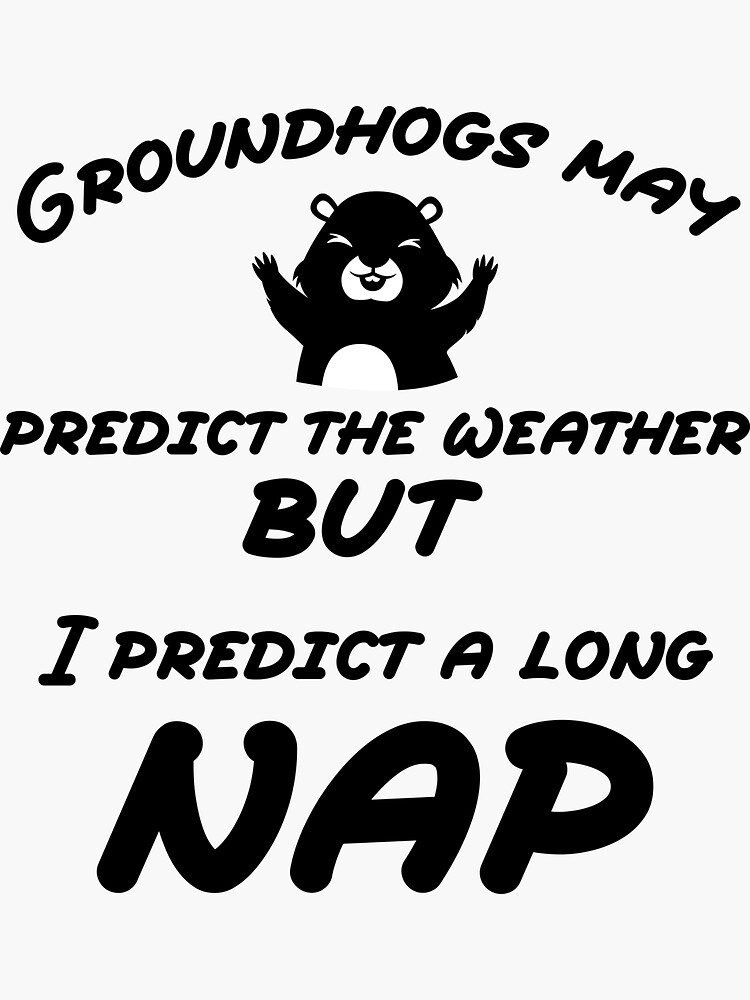This humorous black and white graphic, perfect for social media or office decor, features bold black text on a white background arranged in a playful arc. At the top, it reads, "Groundhogs may predict the weather," followed by an illustration of a cheerful groundhog with its arms up. Beneath the illustration, continuing the text, it declares, "but I predict a long NAP," with "NAP" in the boldest and largest font. The cute, cartoony groundhog adds to the lightheartedness of the message, making it a quirky statement piece for those who enjoy humorous remarks about sleep.